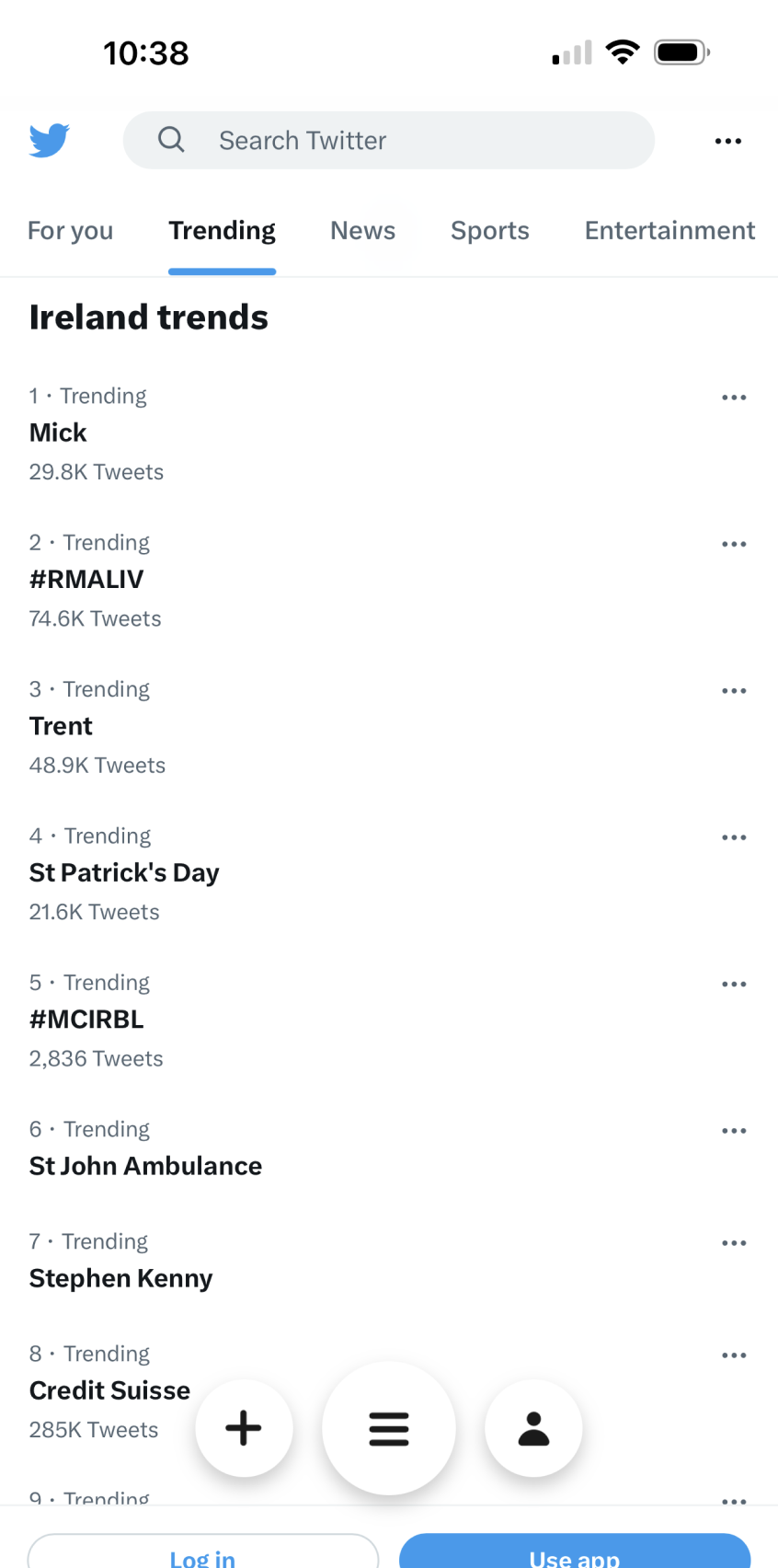Screenshot of a smartphone display at 10:38 AM, showing full signal and battery levels. The screen is on the Twitter app, specifically in the "Trending" section, indicated by a blue underline below the "Trending" tab among the options "For You," "Trending," "News," "Sports," and "Entertainment". 

Under "Ireland Trends," the top trending topics are listed as follows:
1. "Mick" with 29,000 tweets.
2. "#RMaliv" with 74.6K tweets.
3. "Trent" with 48.9K tweets.
4. "St. Patrick's Day" with 21.6K tweets.
5. "McCurble" with 2,836 tweets.
6. "St. John Ambulance" (no tweet count available).
7. "Stephen Kenney" (no tweet count available).
8. "Credit Suisse" with 285K tweets.

Additional icons at the bottom of the screen include a plus sign, three horizontal lines, and a person icon.